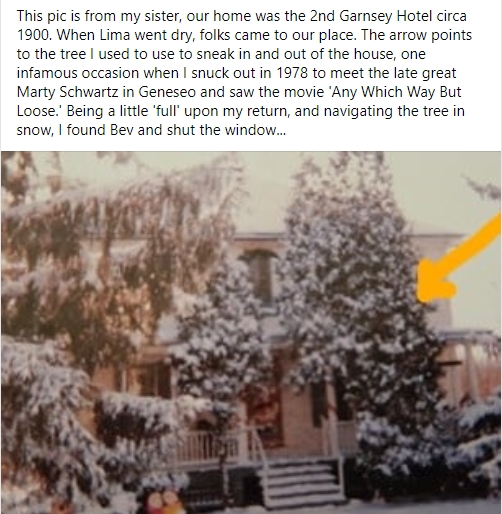The image captures a historical, somewhat faded and blurry two-story white house, believed to be the second Guernsey Hotel dating back to circa 1900, when Lima went dry and attracted visitors. The house is partially hidden behind several tall, snow-laden green pine trees. In the foreground, snow-covered steps lead to a porch with a white fence. A yellow arrow on the right side of the image points to a particular tree. A detailed caption at the top of the photo narrates a personal story: This tree was used by the author to sneak in and out of the house, including one unforgettable night in 1978. The author snuck out to meet friends, the late great Marty Schwartz and Genisio, to watch the movie "Any Which Way But Loose." Upon returning, slightly inebriated and navigating the snowy tree, the author closed the window behind them. The image was provided by the author's sister.